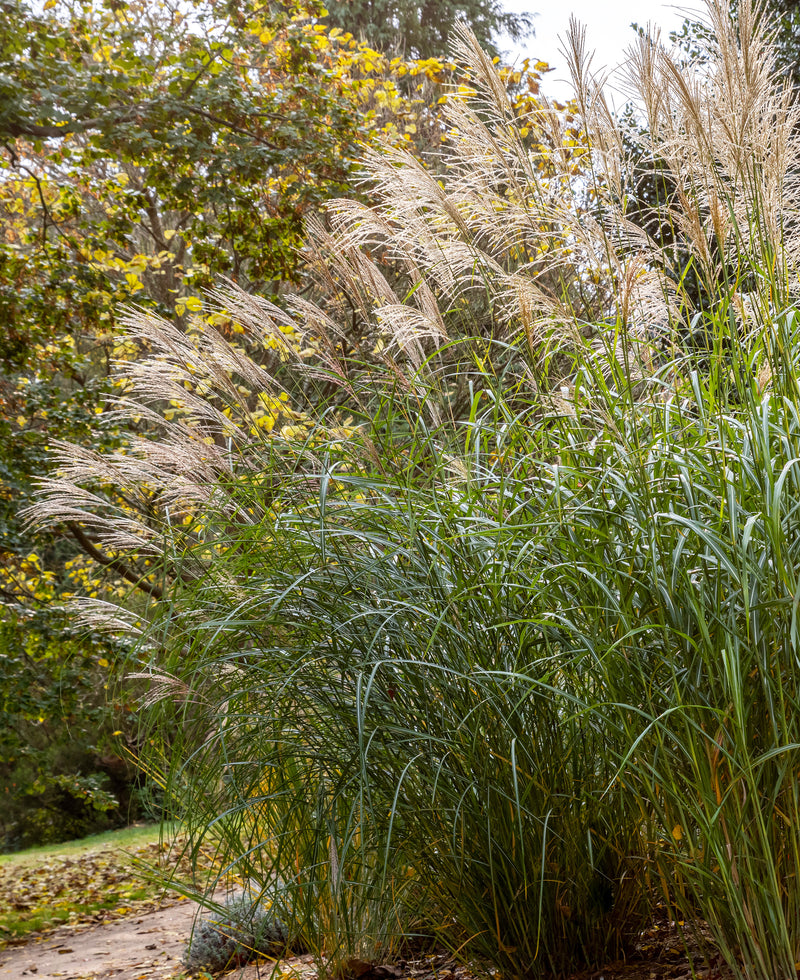This photograph captures a serene outdoor scene prominently featuring tall pampas grass that takes up most of the right side center and top right of the image. The grass, with its long, wispy blooms that are brownish, whitish, and grayish, appears to be gently swaying, pointing toward the upper left, giving the impression of a light breeze on an overcast day. The spindly, curved stems at the bottom right corner exhibit deeper and lighter shades of green, adding texture to the shot. The background is lined with a variety of trees, ranging from deciduous with shades of green and yellow to an evergreen standing further back, suggesting the scene is set in the fall. The bottom left of the image reveals a concrete path bordered by scattered brown leaves on the grass, enhancing the autumnal mood. The sky is a muted gray, complementing the subdued yet rich color palette of the greenery and fallen leaves.